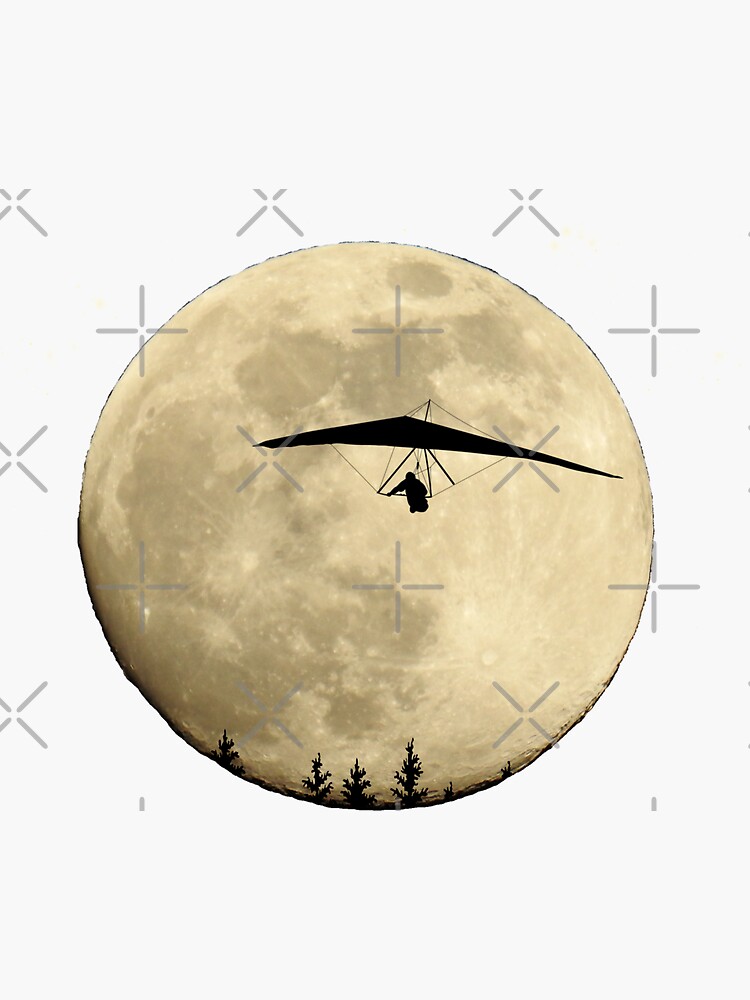The image is a portrait-oriented artwork with a central focus on a large, detailed depiction of the full moon against a white background. The moon, rendered in varying shades of cream and gray to highlight its topography and craters, occupies most of the vertical space. Superimposed over the moon’s center is the black silhouette of a hang glider with an indistinguishable figure, suggesting movement and adding a touch of adventure to the scene. The hang glider is positioned slightly towards the top right of the moon. At the very base of the moon, the dark silhouettes of several pine trees or evergreen tops are visible, creating a sense of depth and grounding the celestial scene. Overlaying the entire image are numerous gray X’s and + signs, subtly blending into the background and adding a textured, almost watermark-like effect. The overall composition evokes a dreamlike and serene quality, combining elements of nature and human exploration in a minimalist yet detailed visual narrative.